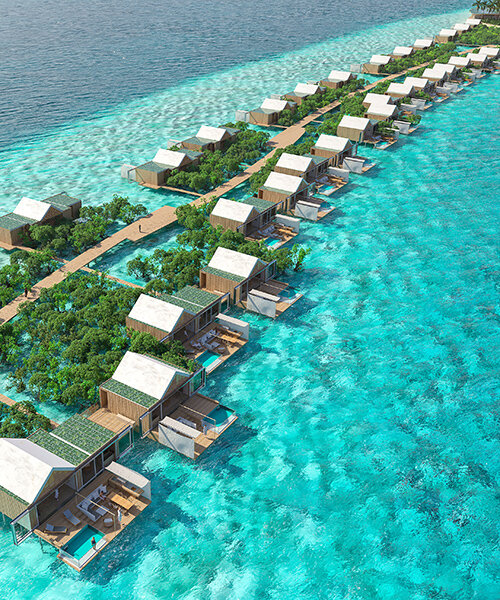This is an aerial photograph capturing a luxurious resort town or fancy hotel getaway featuring a multitude of overwater cabanas situated atop a clear, aqua-colored ocean. The scene is adorned with greenery, including trees and vibrant green bushes, providing a lush backdrop for the floating cabins. The image depicts a thin wooden platform running from the left center of the frame to the top right, with narrow wooden docks extending at regular intervals, each dock flanked by two identical wooden cabanas. These cabanas feature white, sloped roofs with flat green sections next to the walkways. Each cabana boasts an outdoor seating area with white patio furniture and its own private, bright blue swimming pool. The sunny and bright ambiance of the photograph, with its clear skies, suggests a midday setting. The cabanas are fairly close together, creating an intimate yet opulent atmosphere, reminiscent of resorts found in Bali. The abundance of greenery amidst the water, though unusual, adds a touch of surreal beauty to the scene, which might hint at AI generation.